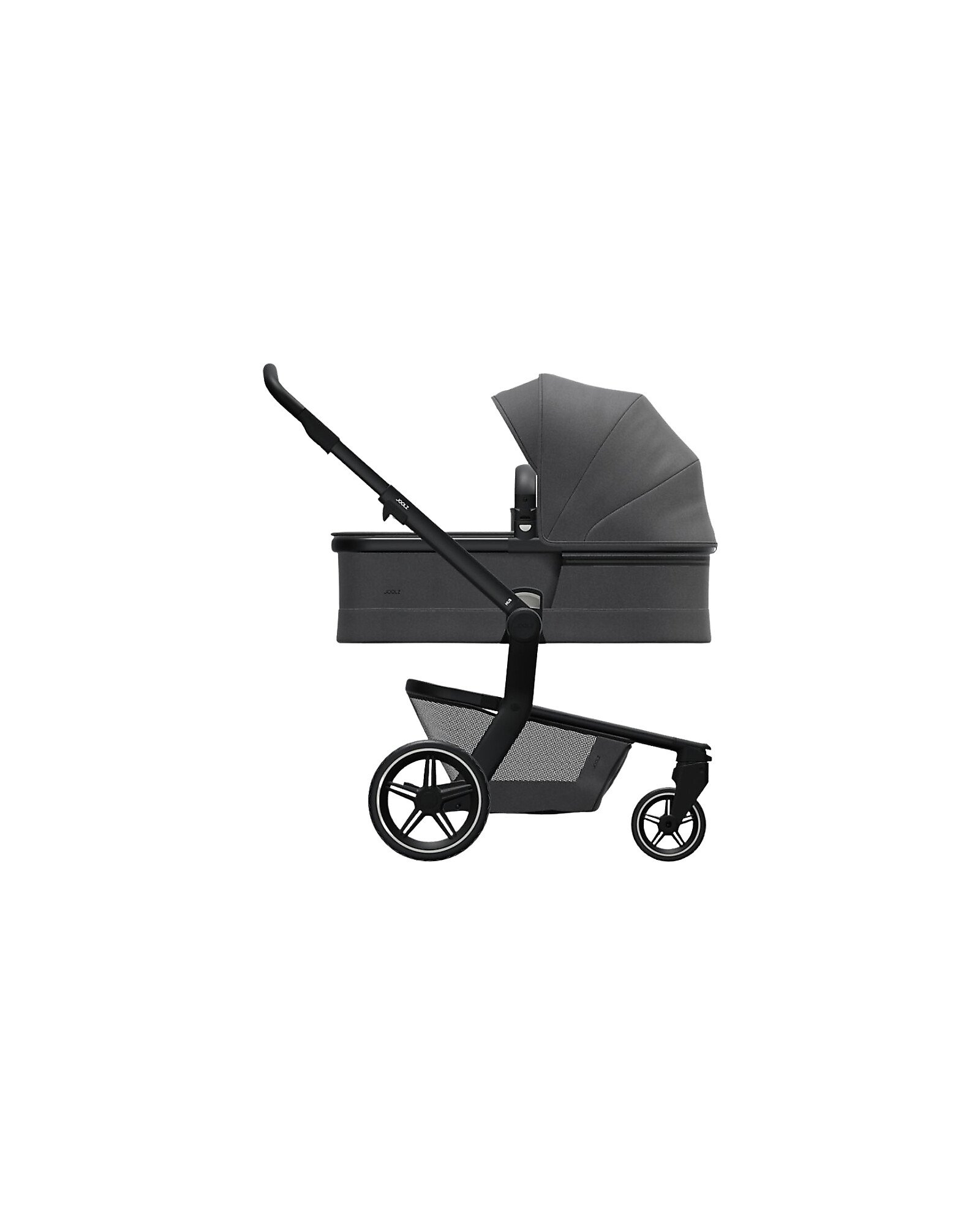This image features a detailed side profile of a baby buggy with a dark gray and black color scheme. The buggy has a distinctive three-wheel design, with the front wheel being smaller in diameter compared to the larger back wheels. Each wheel features five spokes and is black in color. The handles and hardware parts are also black, and the handle extends out from the back of the buggy at a 45-degree angle. The hood, which is fully deployed, covers the front half of the buggy and is dark gray. Beneath the main seating area is a gray netted storage compartment attached to the frame, providing additional space to carry items. The background of the image is plain, set against a white screen.